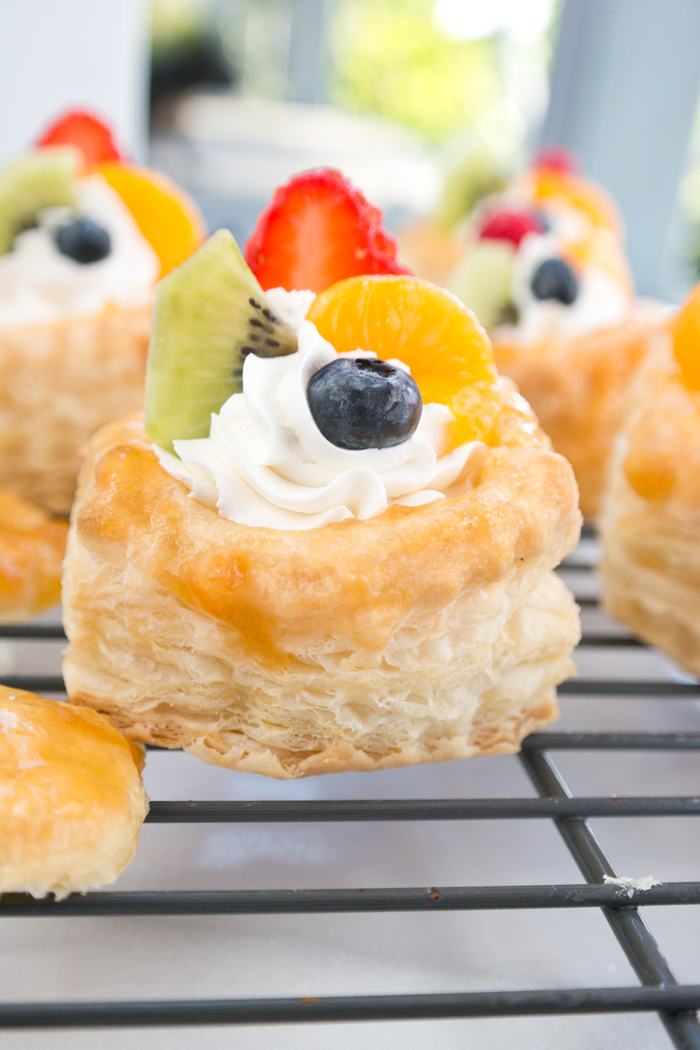This is a detailed close-up image of a delightful pastry resembling a fluffy, puffy biscuit or crumpet. The pastry is a light, off-white to very light brown color, indicating layers of flaky, risen dough that look sweet and delicious. Atop this pastry is a generous swirl of white cream, possibly whipped cream, cream cheese, or icing. Nestled into this creamy topping are several fresh, colorful fruit pieces: a whole blueberry, a strawberry slice, a piece of light green kiwi, and a segment of tangerine or mandarin orange. The pastry sits prominently on an oven rack, with several similar treats blurred in the background, suggesting a collection of these deliciously decorated pastries. One partially-eaten pastry is also visible, adding a candid touch to the scene. The fruits on each pastry are carefully arranged, making the overall presentation both appealing and mouthwatering.